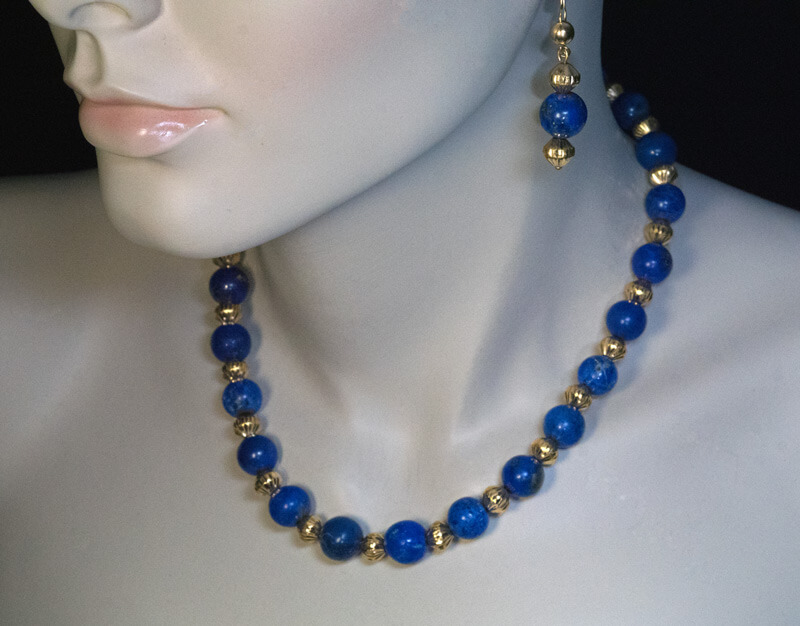This detailed close-up image showcases a photorealistic mannequin adorned with a matching blue and gold jewelry set. The fair-skinned neck and face of the mannequin are highlighted by distinctly pink, glossy lips and subtly tinted cheeks. The main focus is on the intricately designed jewelry: the necklace, a choker of approximately 16 inches, features alternating blue and gold beads meticulously interwoven around the neck. Complementing the necklace are dangling earrings that cascade from the earlobes, mirroring the same blue and gold bead pattern—starting with two gold beads linked by a chain, followed by a blue bead and another gold bead. The mannequin's lifelike features, enhanced by a possible porcelain finish, provide a modern and elegant display, perfect for showcasing the jewelry's vibrant colors and design. The setup is devoid of any clothing, further emphasizing the delicate and intricate craftsmanship of the jewelry set against the mannequin's smooth, polished surface.